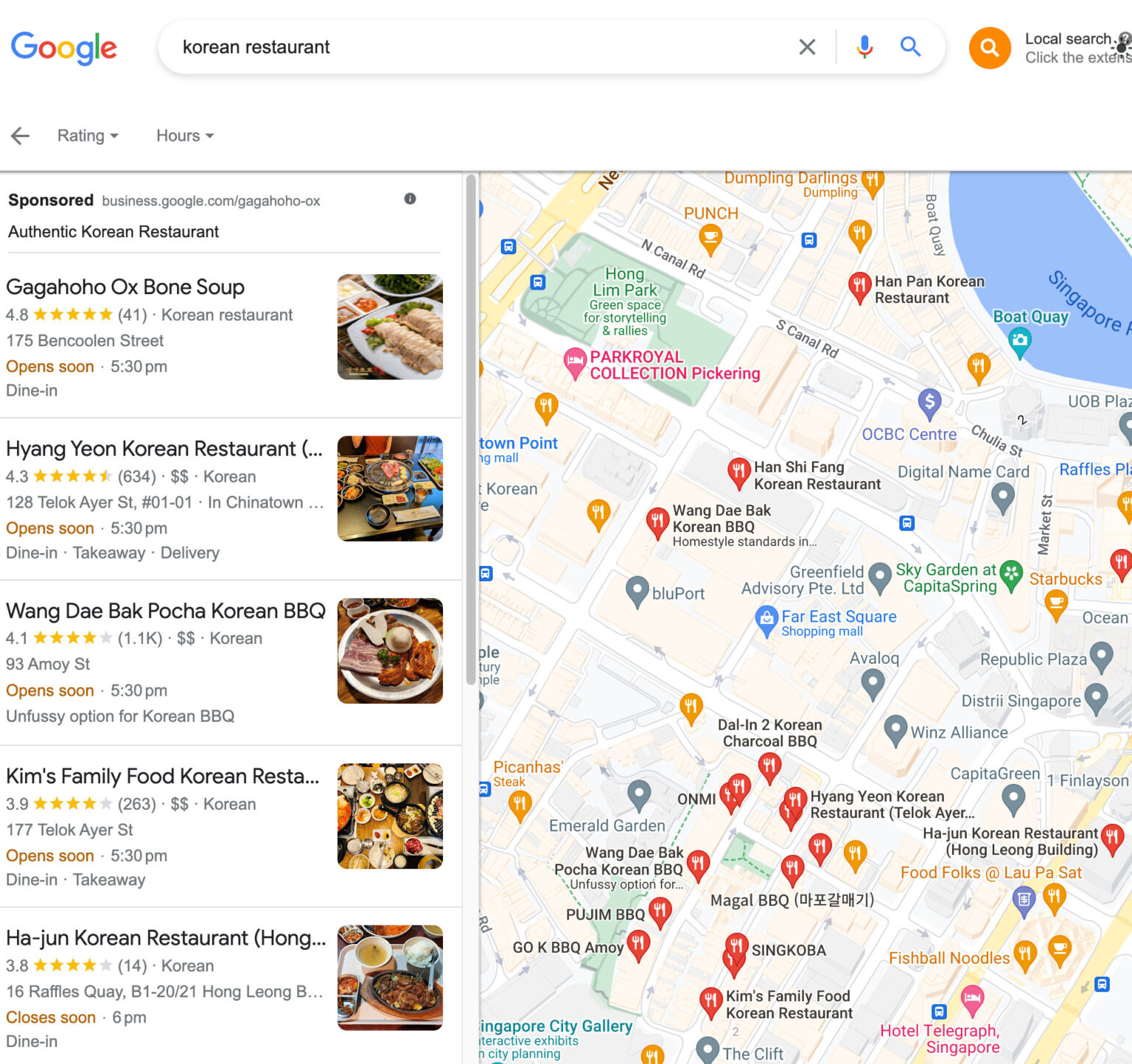This image depicts a detailed Google search results page for Korean restaurants, featuring a prominent map with numerous colorful indicators in yellow, red, and gray, representing various dining options. On the right side of the map, a list of Korean restaurants is organized with noteworthy details. Highlights include Gagahoho Ox Bone Soup with a stellar 4.8-star rating and set to open soon, Hyang Yon Korean Restaurant with a 4.3-star rating also scheduled to open soon, and Wong Daebak Pokka Korean BBQ with a 4.1-star rating. Additional listings include Kim's Family Food Korean Restaurant with a 3.9-star rating and Ha Jun Korean Restaurant at 3.8 stars. The map is cluttered with blips, indicating the density of Korean dining venues. To the left of the map, textual information includes the Back Arrow button, user ratings, hours of operation, and some sponsored business snippets. The bottom of the image prompts users to explore further by clicking the "Experience" button.